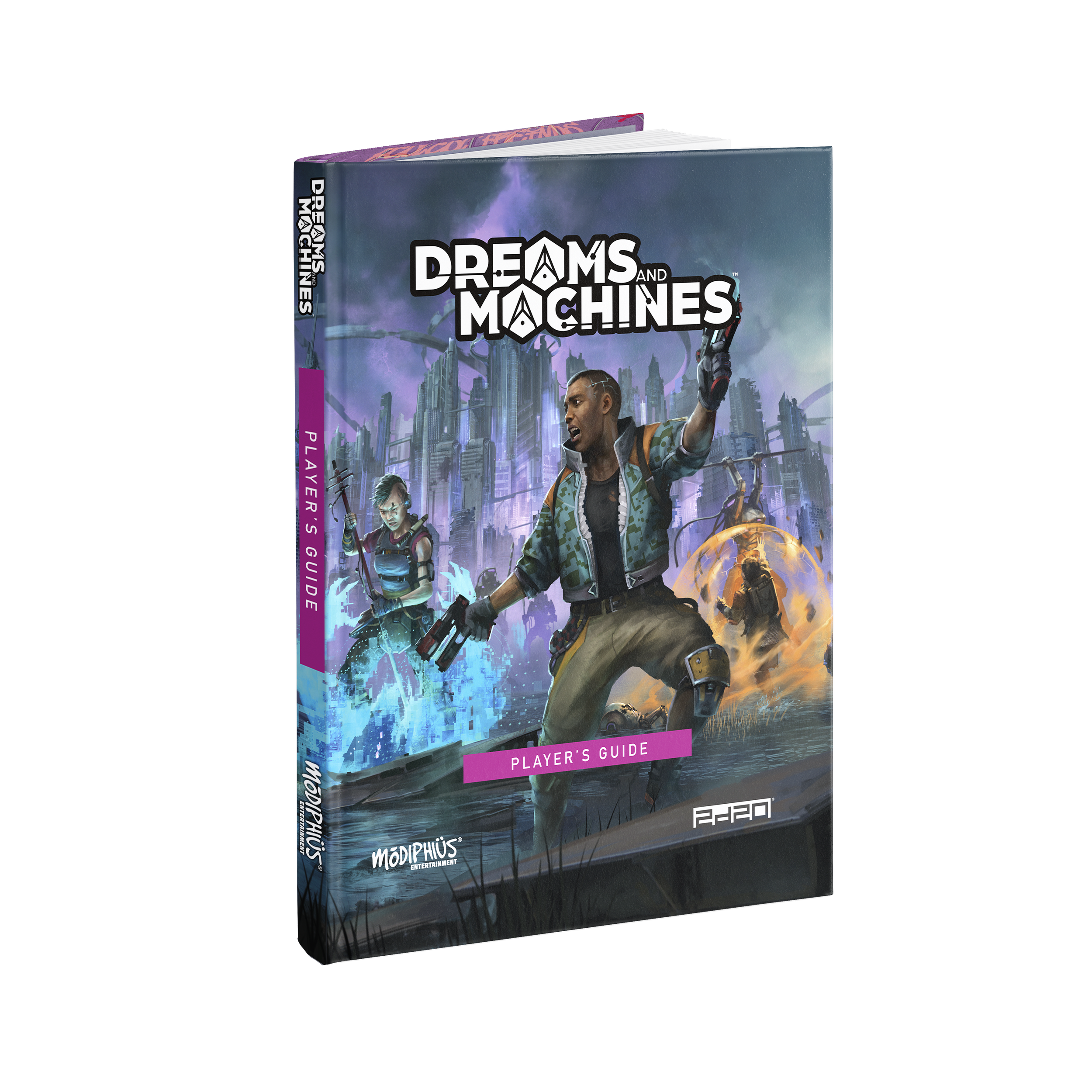The image depicts a standing, slightly open book, with the titles "Dreams and Machines" across the top and "Player's Guide" at the bottom. The cover features an illustration with a vivid sci-fi fantasy theme. Prominently, a black man stands at the forefront wearing a blue and green jacket, gray pants, a black t-shirt, and gray gloves, clutching a pistol. Behind him is a white man donned in an armored vest with a purple shirt, black pants, holding a large stick or sword. The background depicts an apocalyptic city skyline with explosions and fire. To the left, a figure emanating blue and orange energy, possibly a woman with a sword, stands amidst the chaos. The book spine repeats the titles in a white, all-caps font against a violet rectangle and displays the publisher's name, "Modiphus", at the bottom.